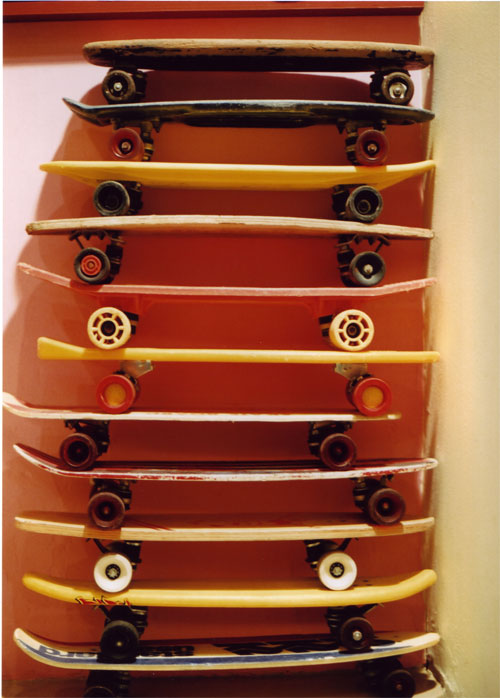The image showcases an assortment of 11 skateboards stacked vertically against a white wall with an orange, shiny backdrop casting shadows. Each skateboard exhibits its own unique characteristics, with a mix of vintage and possibly newer designs. The skateboards display a variety of color schemes, including blue and white, yellow, pink, unpainted, faded red, and black, some bearing visible lettering. The wheels also vary, featuring shades of orange, white, red, and black, with conditions ranging from pristine to heavily worn. The arrangement, starting from the bottom, includes a blue and white skateboard, followed by a yellow one, then an unpainted board, a faded red one, another white, another yellow with perfect wheels, a pink one also with well-preserved wheels, a very faded brown one with mismatched wheels, another yellow one with wheels in poor condition, a faded black skateboard with replaced red wheels, and finally, at the top, a black skateboard showing significant wear and tear.